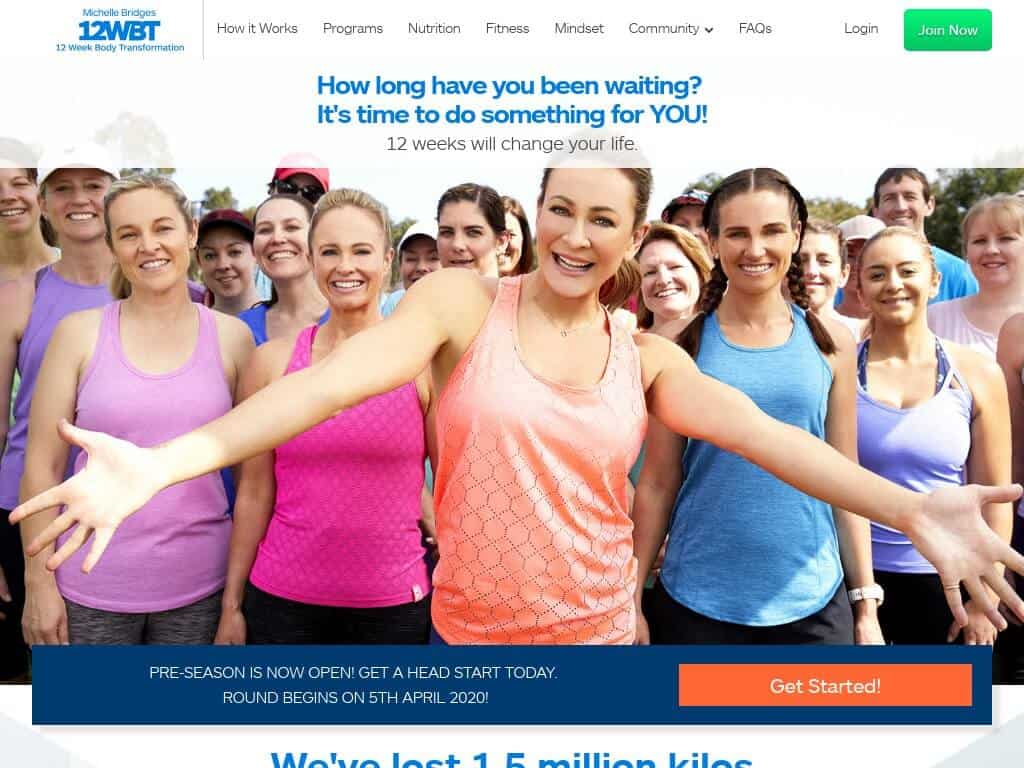This is a detailed screenshot of a web page, likely displayed on a tablet or laptop. The central image features a slender white woman with her arms stretched out and wearing her hair pulled back into a ponytail. She is dressed in a peach-colored tank top adorned with a honeybee design. Surrounding her are approximately 12 women and two to three men, all of whom are white and smiling. The majority of the women also wear their hair pulled back, and some individuals have on caps. Notably, one man in the background is wearing a red cap with sunglasses.

In the forefront, the women are dressed in a variety of tank tops, including colors like dark purple, light purple, pink, blue, and a purplish-blue hue. Above this group, there is a motivational message: "How long have you been waiting? It's time to do something for you. 12 weeks will change your life." Below that, another message reads: "Preseason is now open. Get a head start today. Round begins on 5th April 2020." A prominent orange bar encourages visitors to "Get started."

At the lower section of the screenshot, there's partially visible text indicating an impressive achievement: "We've lost 1.5 million kilos." The top left corner features the brand name "Michelle Bridges" followed by "12 WBT" and "12-Week Body Transformation." The top navigation bar includes categories such as "How it works," "Programs," "Nutrition," "Fitness," "Mindset," "Community" (with a drop-down menu), "FAQs," "Login," and a green "Join now" button.